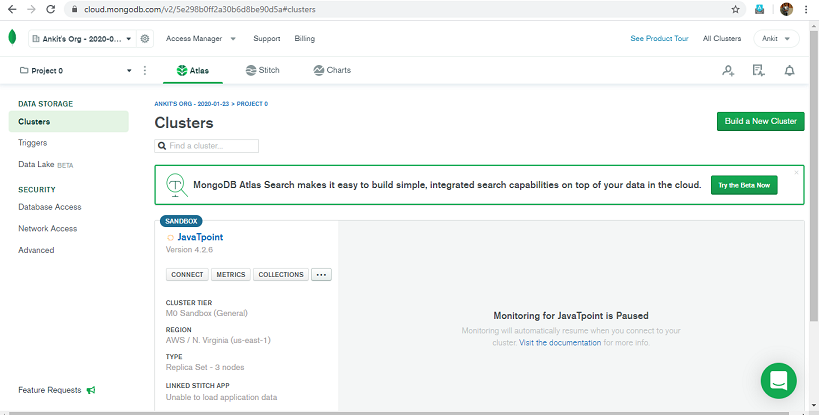This image depicts a screenshot of a cloud management website, specifically at the URL cloudmongodb.com, as indicated in the top-left corner of the browser window. The browser navigation includes a back arrow, forward arrow, and a refresh button to the left, while to the right, there are icons for printing and profile settings.

Below the browser's address bar, the website interface is organized into several sections. On the left sidebar, options listed include file section, Access Manager, Support, and Billing.

Prominently on the right-hand side of the interface, a blue button labeled "See Product Tour" is visible. Adjacent to this are options titled "All Clusters" and another unidentified option.

The website content is divided into three main categories, with "Atlas" being highlighted with a green underline, followed by "Stitch" and "Charts." Beneath this are additional sections. The "Clusters" section features a mini search bar for locating specific clusters and a green button labeled "Build a New Cluster."

Further down, a green rectangle highlights a feature stating, "MongoDB Atlas search makes it easy to build simple integrated search capabilities on top of your data in the cloud." Another green rectangle is positioned to the right.

In the lower section, a heading labeled "Java T-Point" is followed by options such as "Connect," "Metrics," and "Collections," displayed against a white background. Next to this, in a gray background, is the information, "Monitoring for Java T-Point is paused."

On the left-hand side, under a section titled "Data Storage," various categories are listed, although they are not fully detailed in the image.